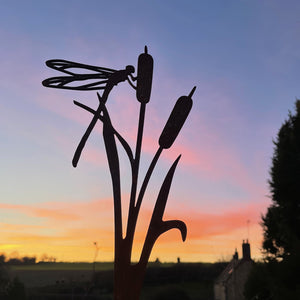The photograph showcases a metallic sculpture of a cattail plant, planted firmly on a grassy field. The intricate sculpture features two cobs and leafy structures, perfectly mimicking the appearance of a real cattail. Perched atop one of the cattail cobs is a metallic dragonfly with transparent wings. Both the plant and the dragonfly are captured in silhouette form, giving them a striking pitch-black appearance against the vibrant backdrop.

The sky is awash with beautiful blue and pinkish hues, indicating the time of sunset or sunrise. To the right of the sculpture, a tree can be seen, which appears black against the colorful sky due to the lighting. Additionally, there is a barely visible building and what looks like a fence further to the right. The outdoor setting of the photograph, combined with the artistic elements of the metallic sculpture and the natural beauty of the sky, creates a stunning visual narrative.